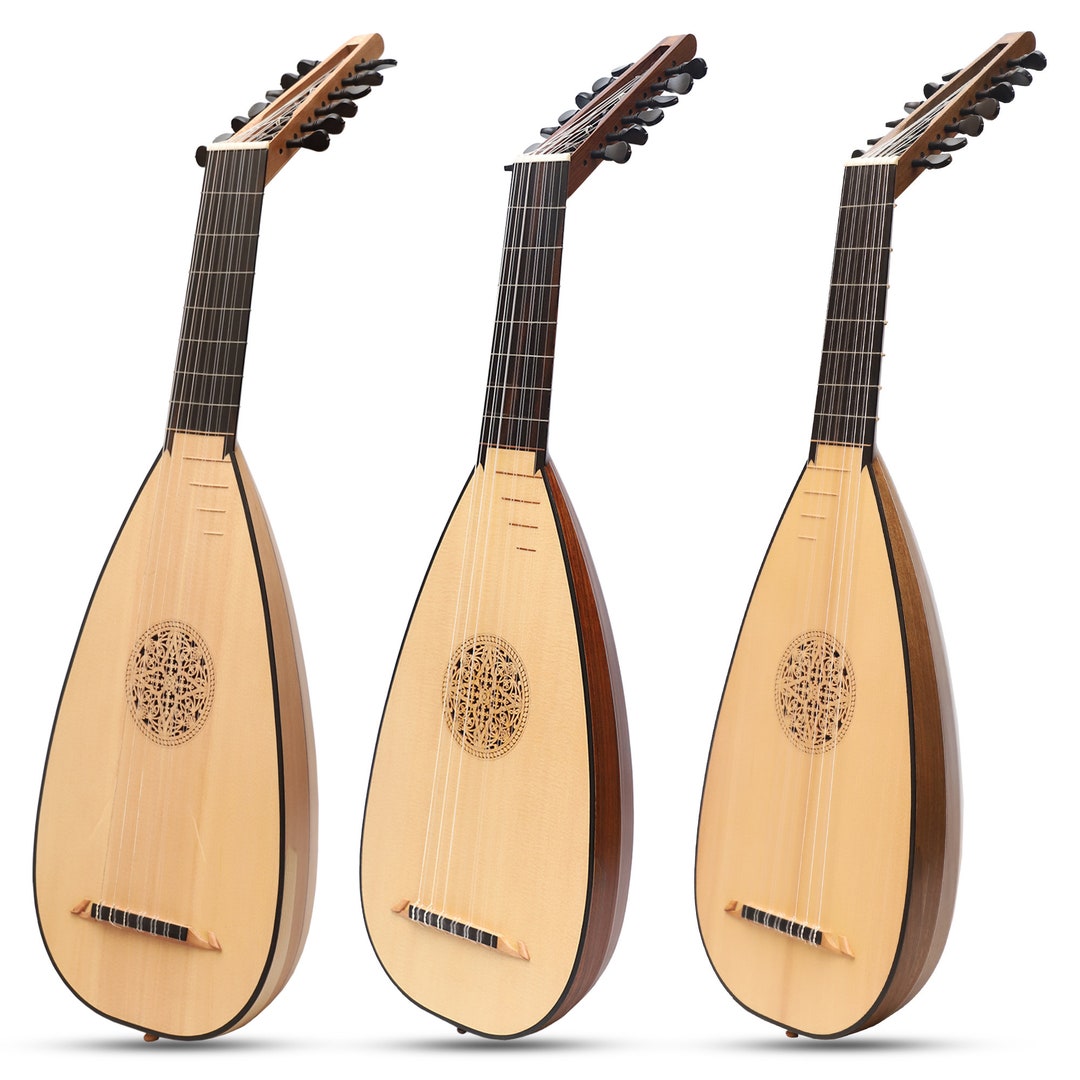This photographic image depicts three identical lutes, classical stringed instruments with roots in the Middle East, displayed against a stark white background. The lutes, laid out in a diagonal formation from left to right, showcase their light brown wooden soundboards. Each lute features a belly crafted from darker wood, contributing to the aesthetic contrast. 

The strings of the lutes stretch across the soundboard, converging near an elaborately carved sound hole, adorned with an intricate geometric pattern. Unlike typical guitars, the necks of these lutes are black and the tuning knobs are positioned at an incline, offering a unique visual disparity with their angled setup. The considerable craftsmanship is evident in the interplay of light and dark woods, lending a sense of depth and texture to the image. Absence of any text keeps the focus solely on the elegant design and details of these exquisite instruments.